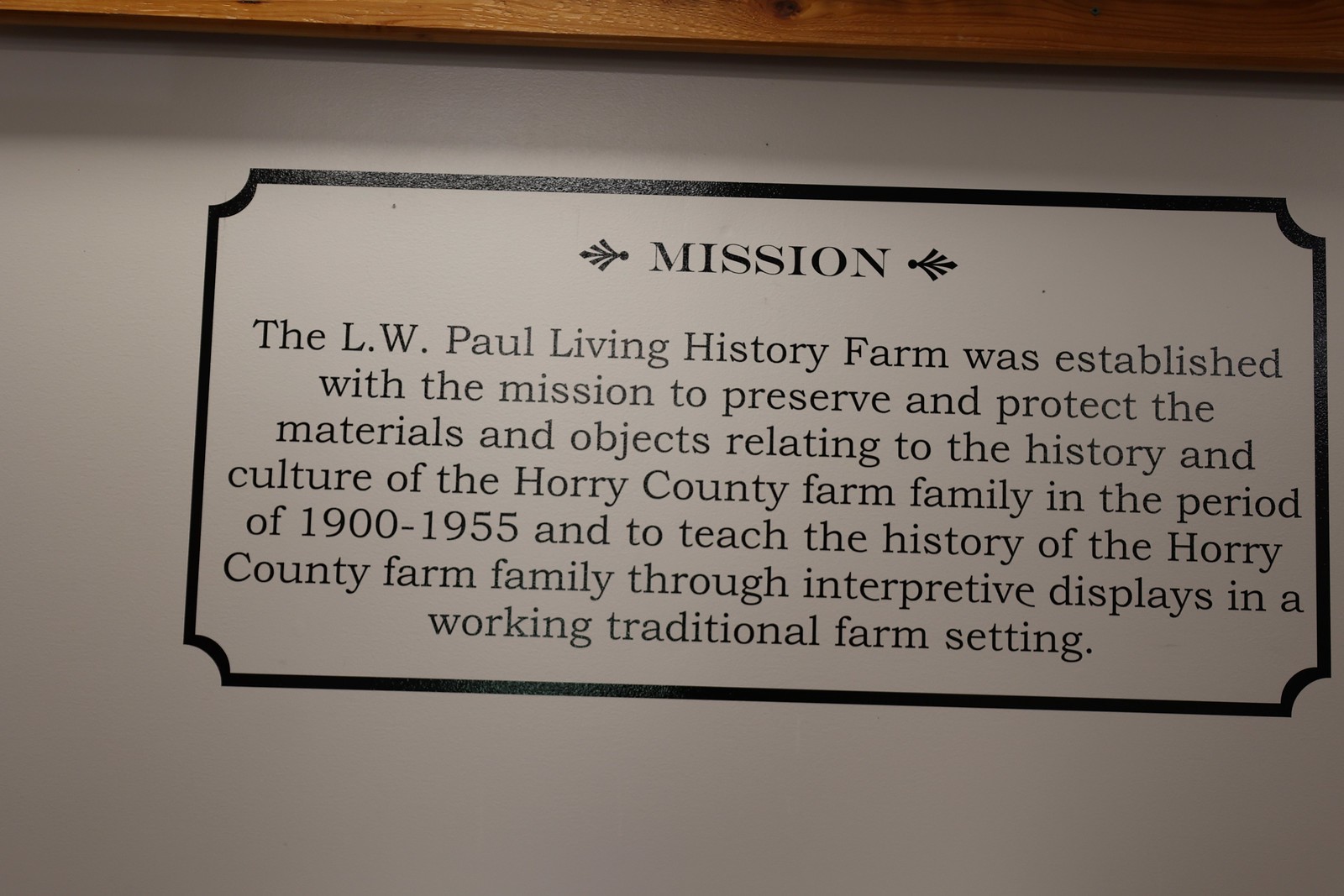The image shows a white background with a wooden area at the top, and a rectangular black outline in the shape of a ticket stub with inward-curving corners. Inside the outline, it reads "Mission," followed by a detailed description. The text explains that the L.W. Paul Living History Farm was established to preserve and protect the materials and objects related to the history and culture of the Horry County Farm Family from 1900 to 1955. It also aims to educate about this history through interpretive displays in a working traditional farm setting. The photographic angle suggests it might be a wall-mounted sign or plaque offering information about the museum's purpose.